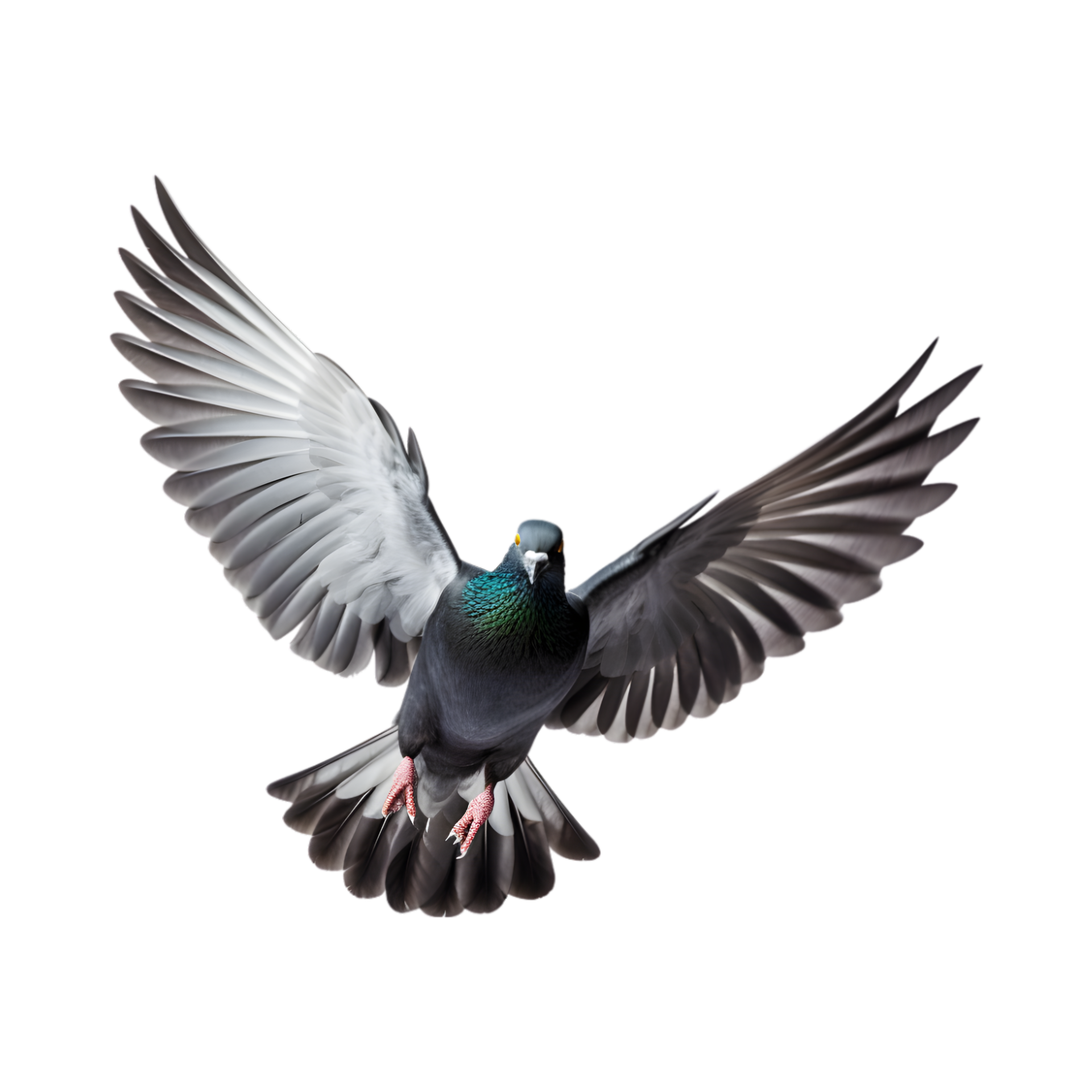This image features an AI-generated cartoon of a bird, likely a pigeon, flying towards the viewer against a stark white background. The pigeon has large, outstretched wings displaying a gradient of colors from light gray to dark gray, with white and black accents on the underside and top of the feathers respectively. The bird's talons, tipped with small claws, are extended downwards and have an orangish-reddish hue. Its short, fanned tail feathers, matching the wing feathers in their gray color, aid its flight. The pigeon’s body is predominantly gray, adorned with subtle iridescent hints of blues, greens, teals, and yellows on its chest. The bird’s eyes are a striking orange, set on either side of its face, which features a light grayish-white beak. Individual feathers are discernible on the wings and tail, capturing a detailed and dynamic depiction of the pigeon in mid-flight.